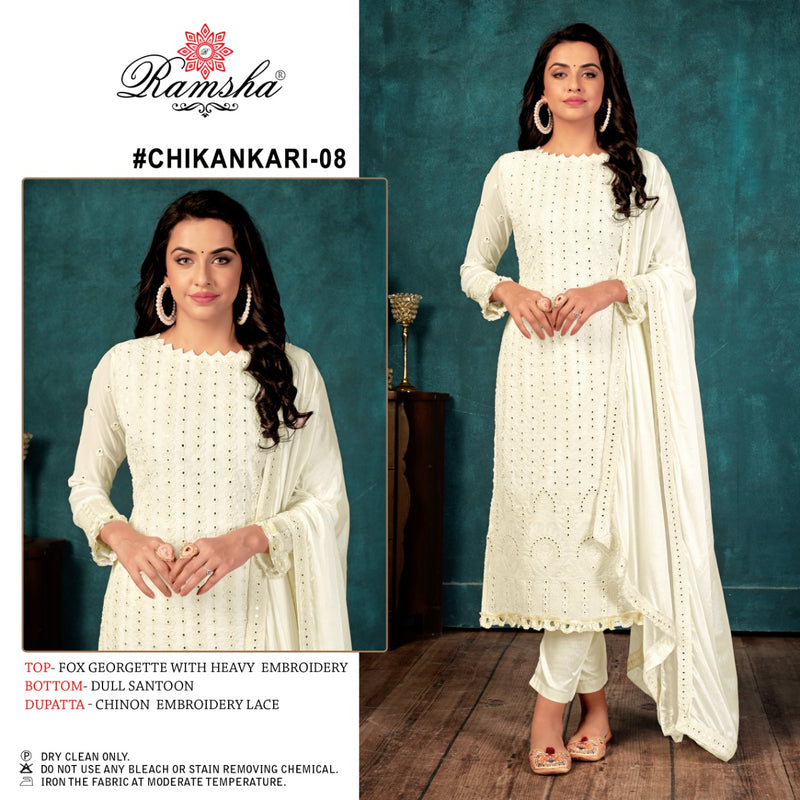The image is a composite of two photographs placed side-by-side, forming a square image roughly six inches by six inches. The left photograph is a cropped, zoomed-in portion of the right photograph, focusing on the woman from her waist up. The background features a greenish-blue painted wall and dark brown wooden flooring. The woman appears to be of Indian descent with light brown skin, long curled brown hair, and a small bindi on her forehead. She is wearing large white hoop earrings, a long-sleeve white tunic adorned with beads, an over-jacket draped over her left shoulder, white pants, and small slippers. She also has two large rings and one smaller ring on her fingers. To the left of the photographs, a red star or flower sits above the name "Ramsha" in black cursive, followed by the designation "#CHIKANKARI08" in black print. Below the smaller image on the left, more text in red and black print provides details about the outfit: "Top" describes "Fox Georgette with Heavy Embroidery," "Bottom" is identified as "Dul Santun," and "Dupatta" features "Chinan Embroidery Lace." The care instructions specify "dry clean only, do not use any bleach or stain removing chemical, iron the fabric at moderate temperature." Additionally, a wooden table appears in the background on the left side of the larger photograph, adorned with an antique object.